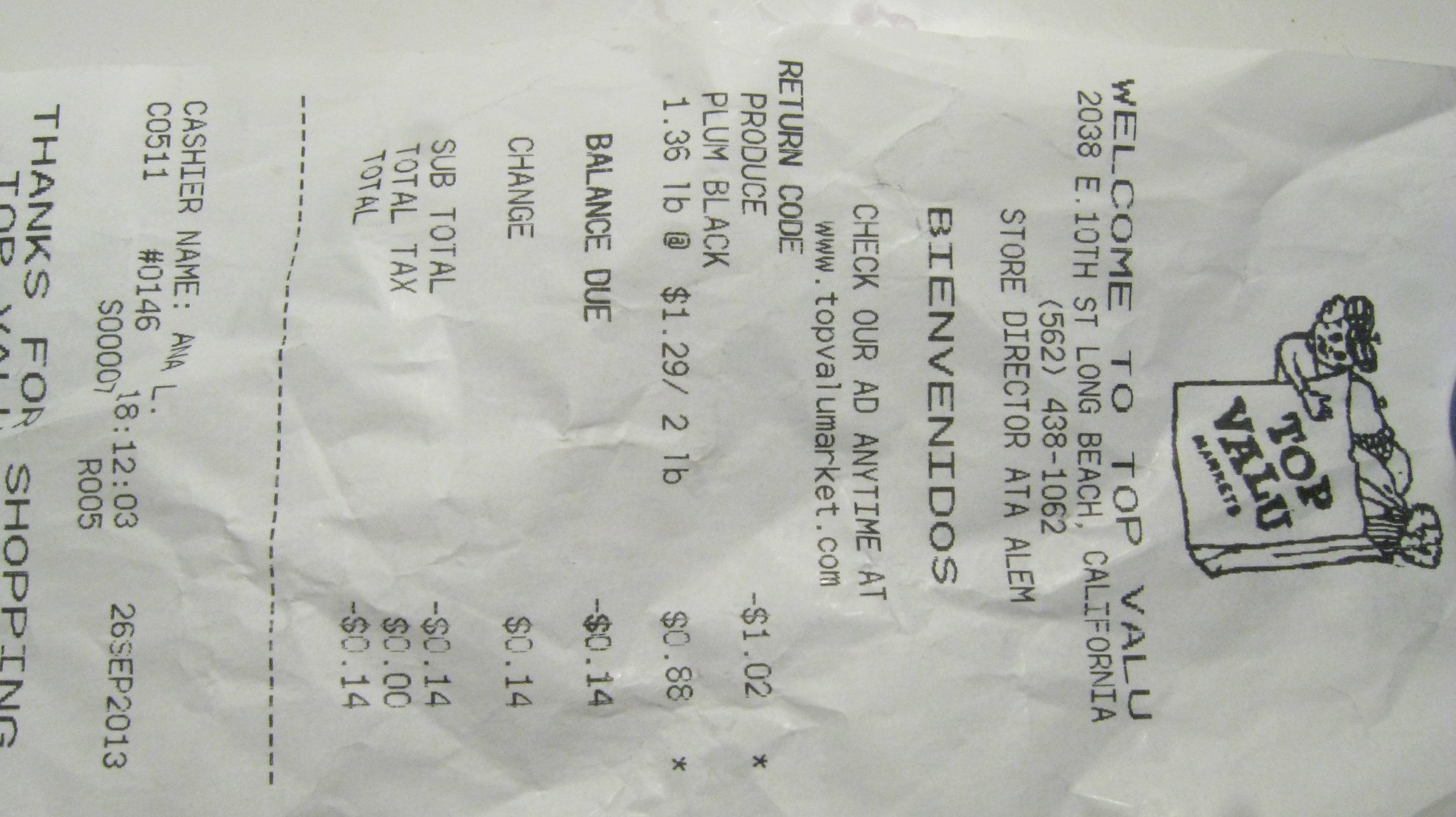The image depicts a wrinkled white receipt with black text, placed on its side with the top oriented to the right and the bottom to the left. At the top of the receipt, there is a logo for “Top Value Markets,” featuring a shopping bag filled with fruits and vegetables. A person wearing a beanie hat is depicted clinging to the side of the bag. Below the logo, it reads “Welcome to Top Value” and includes the store’s address, phone number, and the store director's name. The text also features a welcoming message in Spanish, "Bienvenidos," followed by an invitation to "Check out our ad anytime" with the store's website listed. Subsequent sections of the receipt list the purchased produce items along with their prices, the total amount spent, and the cashier's name. Towards the bottom, a series of numbers, including the date "26 September 2013," is printed. The receipt ends with a "Thanks for Shopping" note, though some text beneath it is partially cut off and unreadable.